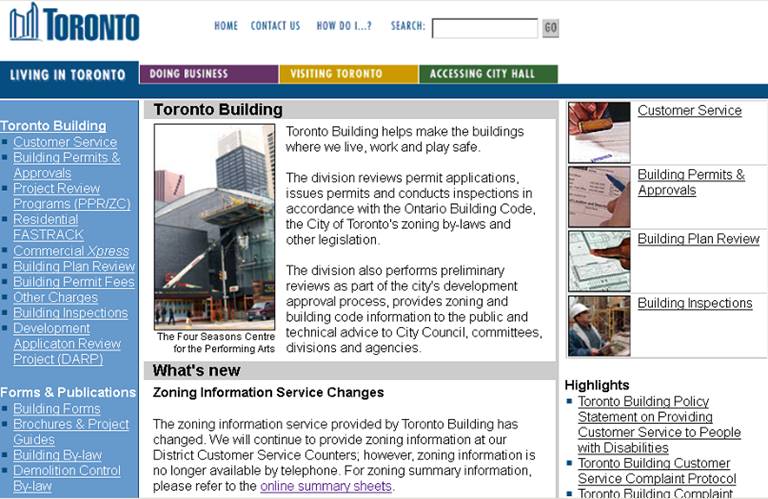The City of Toronto's official website showcases an array of resources and information for residents, businesses, and visitors. In the top left corner, the site is branded with "Toronto" alongside a blue line drawing of the city's skyline on a white background. The website's header features navigation links for "Home," "Contact Us," "How Do I," and includes a search box with a "Go" button.

Currently highlighted under the blue tab titled "Living in Toronto," the page details the Toronto Building program. This division is dedicated to ensuring the safety of buildings used for living, working, and engaging in recreational activities. They handle permit application reviews, issuance of permits, and conduct inspections compliant with the Ontario Building Code, City of Toronto Zoning Bylaws, and other pertinent legislation. Moreover, the division offers preliminary reviews for development approvals, public zoning and building code information, and technical advice to city council committees and divisions.

Central to the page is a photograph of the Four Seasons Centre for the Performing Arts, enhancing the visual appeal of the site. Alongside, there are multicolored tabs for "Doing Business," "Visiting Toronto," and "Accessing City Hall."

On the left-hand side of the page, there is a comprehensive menu featuring links to customer service, building permits and approvals, project review programs, Residential Fast Track, Commercial Express, building plan review, fees and charges, inspections, development application reviews, and various forms and publications. On the right, a separate list of pictorial links offers quick access to customer service, building permits and approvals, building plan reviews, and building inspections. Additionally, a highlights section is positioned at the bottom right, summarizing key information and updates.